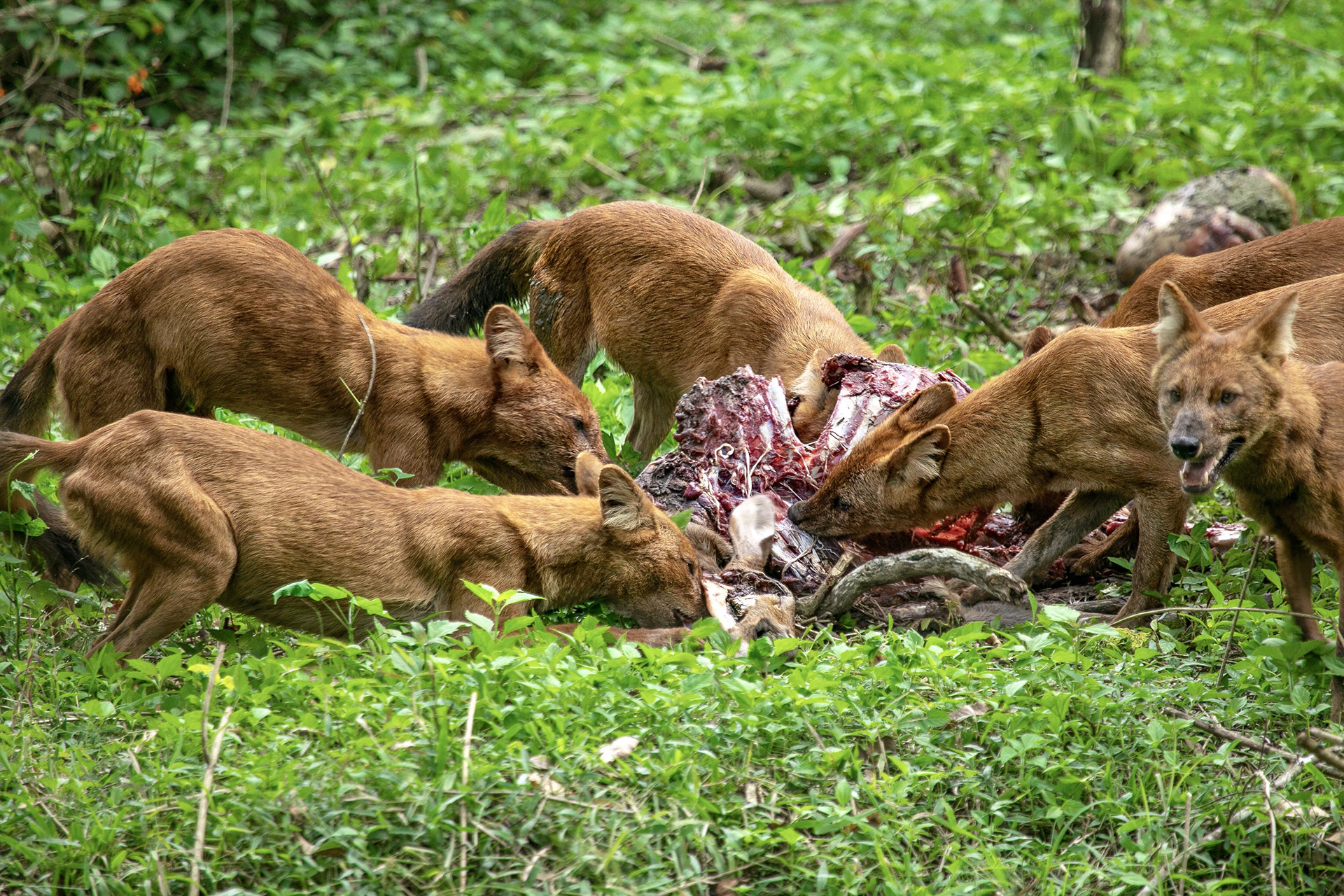In the image, a pack of six coyotes is gathered around a largely unidentifiable carcass, feasting on its remains. Positioned on unkempt, brushy grass resembling a woodland floor, the setting appears lightly wooded with a small tree trunk visible in the background, lending an open and somewhat natural feel. Five of the coyotes are bent over, engrossed in feeding, while the one closest to the viewer on the right stands alert, looking slightly downward to the left. The scene is likely captured during daytime, though not particularly sunny, highlighting the coyotes' brown, healthy-looking fur. The carcass itself is a disarray of purple, red, and white hues, situated at the center of this vivid depiction of wildlife.